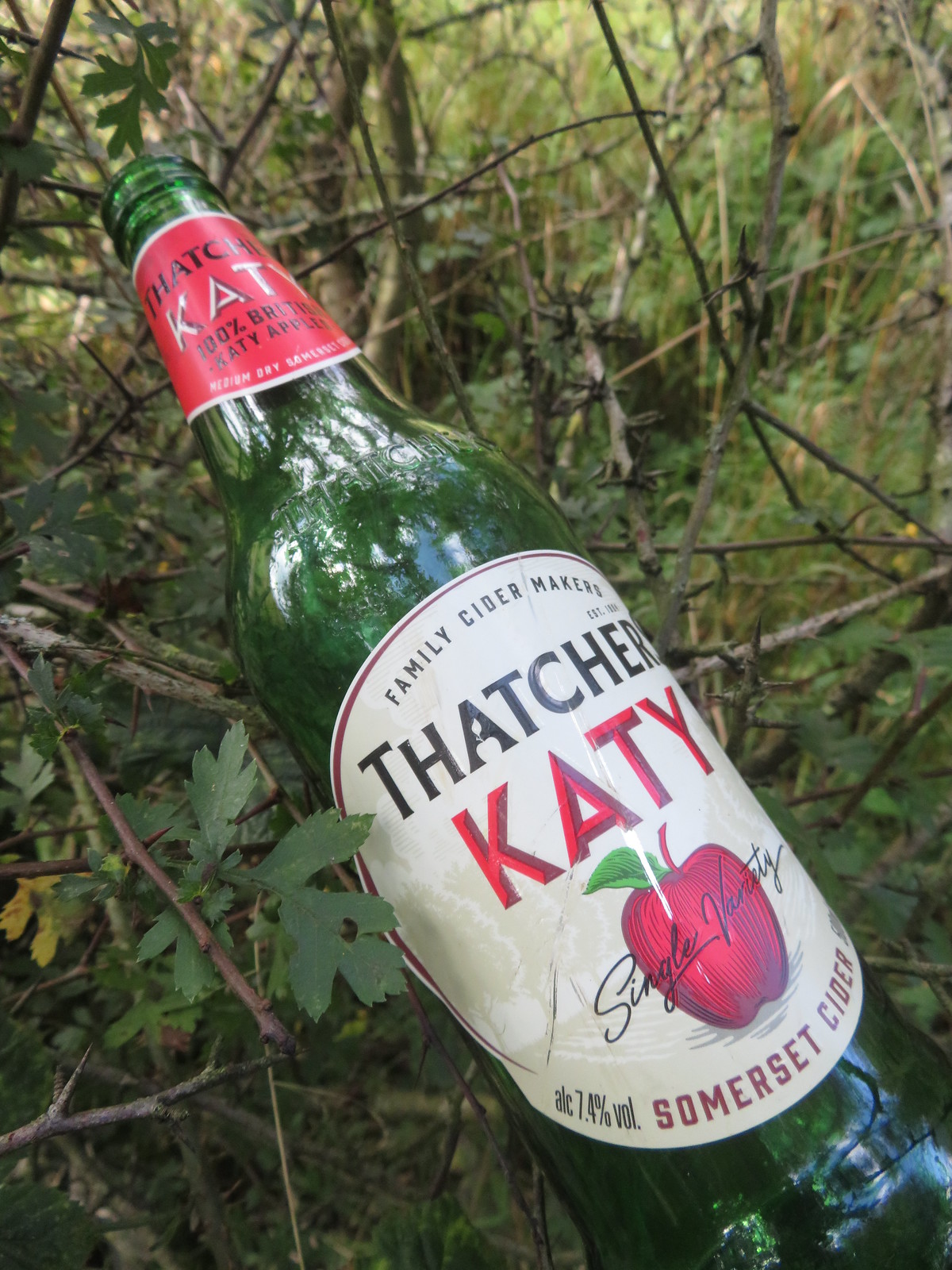This color photograph, featuring a green glass bottle of Thatcher's Katy Apple Cider, is set in a natural backdrop of green grass, twigs, and leaves. The bottle, positioned at an angle with its neck pointing toward the top left corner and its base toward the bottom right, is uncapped and empty. At the top of the bottle is a red necker label with gold lettering that reads "Katie." The bottle’s main label is an oval white background with intricate details: at the top, in small black letters, it says "Family Cider Makers"; below that, in prominent red capital letters with a gray drop shadow, is the name "KATY." Beneath the name is a line art illustration of a red apple with a green leaf and a black script caption, "Single Variety." Along the bottom edge of the label, in all red caps, are the words "Somerset Cider." Additionally, there is a numerical detail, indicating an alcohol content of 7.4% by volume. The photograph is oriented in portrait mode and showcases a high degree of realism, typical of product photography, accentuating the cider bottle amid its lush and rustic surroundings.